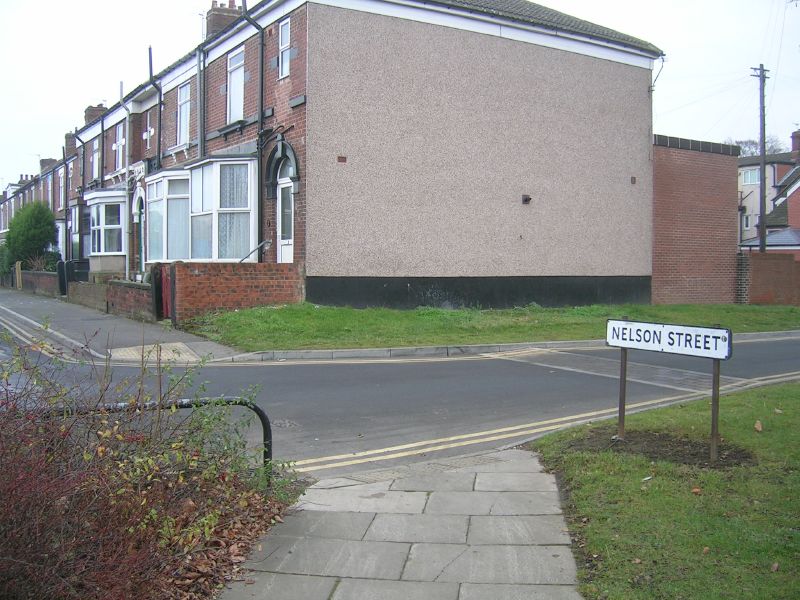The image depicts a stretch of two-story row houses on Nelson Street, viewed from across a small paved road lined with yellow lines and flanked by green grass and bushes. The houses are uniform in appearance, stretching linearly into the distance, and characterized by white bay windows and beige brick facades. A sign to the right of the road reads "Nelson Street" in black letters on a white background. In the foreground, there is a paved sidewalk made of horizontal concrete pieces leading towards the road. The scene is framed by scattered leaves and telephone lines overhead, with the setting under a plain white sky, enhancing the typical suburban environment. The view is taken from a ground-level perspective, capturing the residential street in a realistic, photographic style.